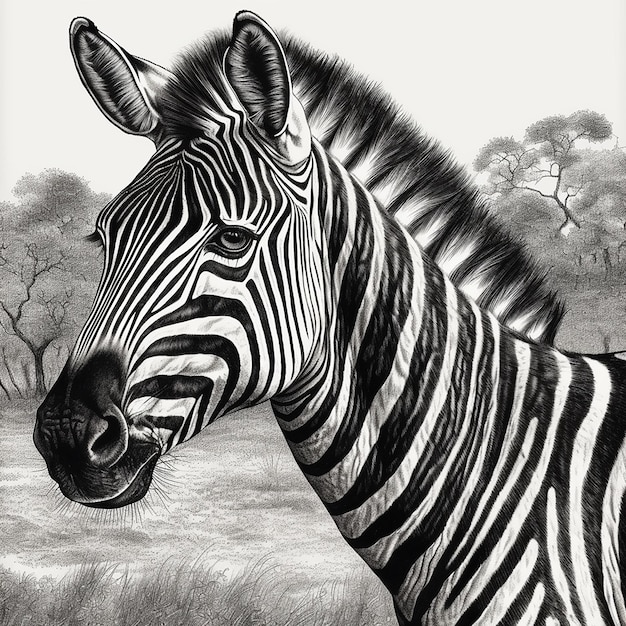This is an intricately detailed black and white pencil drawing of a zebra's head and neck, likely digitally generated. The zebra faces left, displaying its striped mane, dark eye, and a snout with faint whiskers. The ears are prominently framed with fur on the inside and the fuzzy muzzle adds to the textured detail. The background showcases a savanna scene with grasses in the foreground and trees further back, both shaded in gray tones. The sky, depicted in a subtle light gray, provides a neutral contrast, enhancing the outdoor, daylight setting. The overall expression of the zebra hints at a subtle sadness, emphasized by its glossy, somber eye. This artwork captures the serene beauty of the zebra in its natural habitat with impressive detail on the fur, stripes, and surrounding environment.